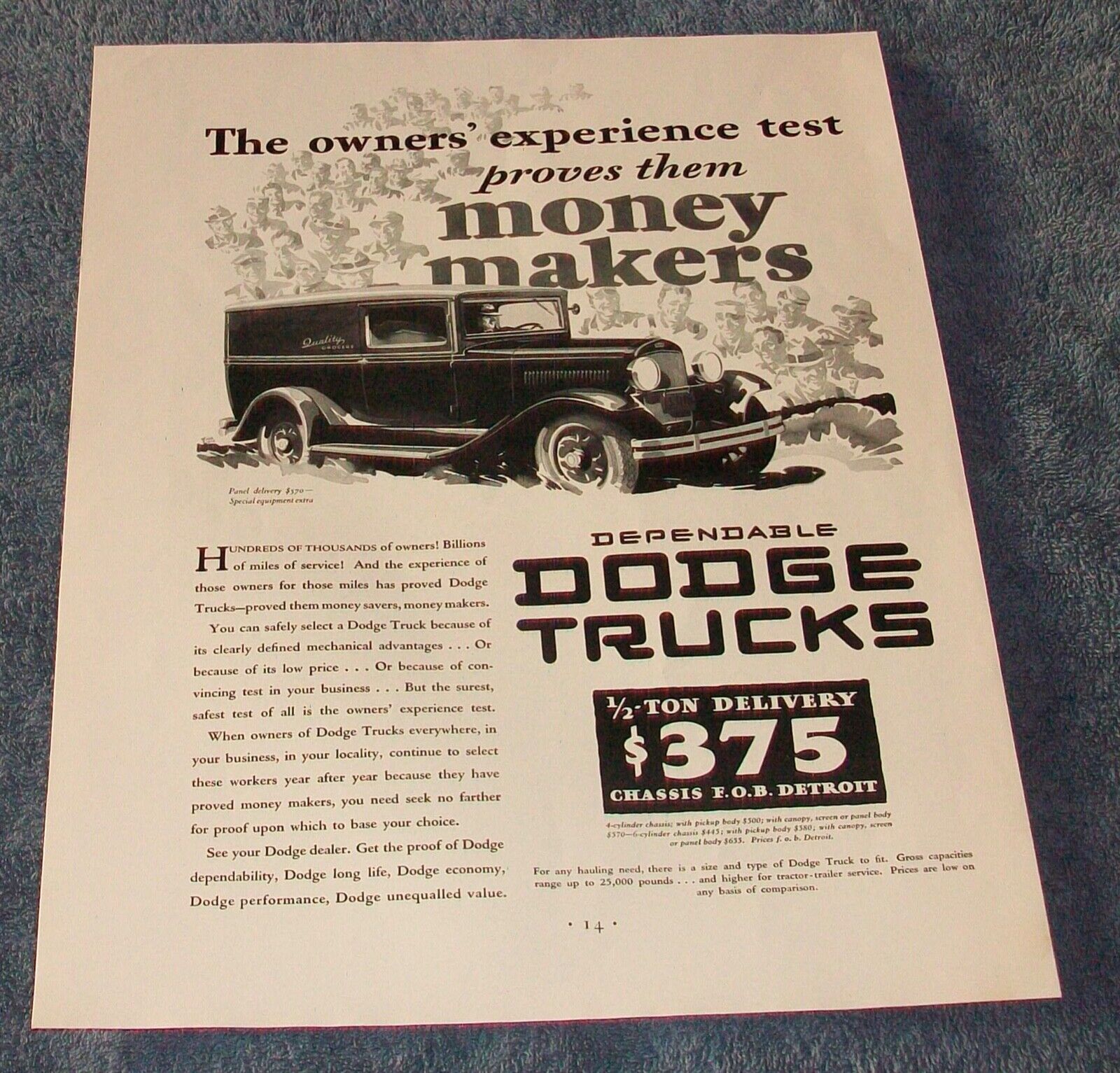This image features a vintage owner's manual, weathered and discolored to a tan hue, placed atop a dark blue rug. The cover prominently states, "The owner's experience test proves them money makers," accompanied by an image of a 1930s Dodge vehicle. A line of men, fading into the background, is visible on the right side of the image. Below the main title, in black lettering, the text reads, "Dependable Dodge Trucks, 1.5 ton delivery, $375, chassis FOB Detroit." While additional text appears next to and beneath these details, it is too small to be legible. The page number 14 is marked at the bottom.